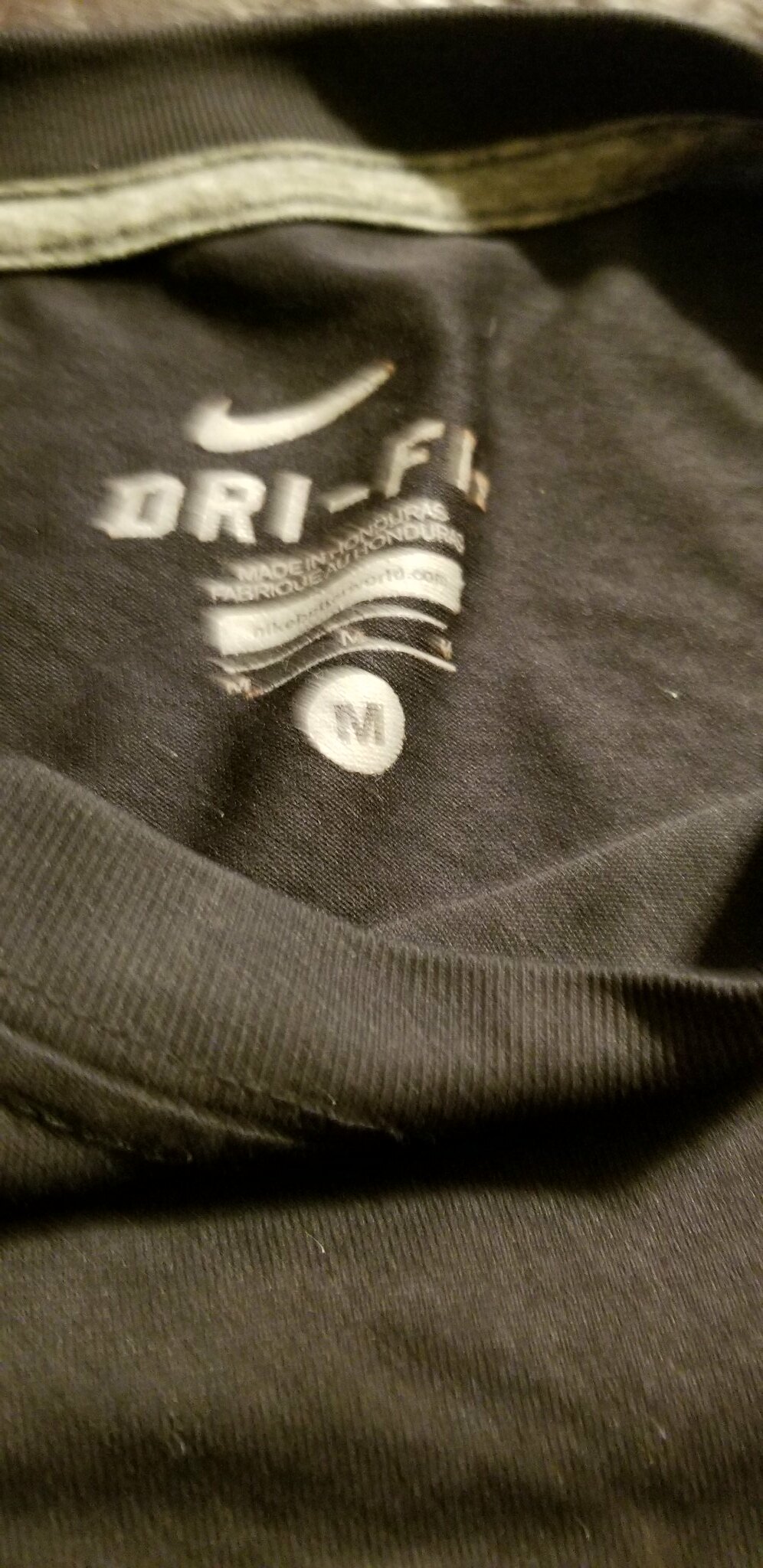This image features a partially out-of-focus, grayish-black t-shirt with a rounded neckline. The visible portion of the shirt reveals a label located near the neck area. The label prominently displays the iconic white Nike Swoosh logo, followed by partially legible text that appears to include "DRI-FIT," indicating it is a moisture-wicking Dry Flex shirt. Though blurred, the label text suggests the shirt is made in Honduras. Additionally, a white circle with an "M" designates the shirt's size as medium. Due to the image framing, it is unclear whether the shirt has long or short sleeves.